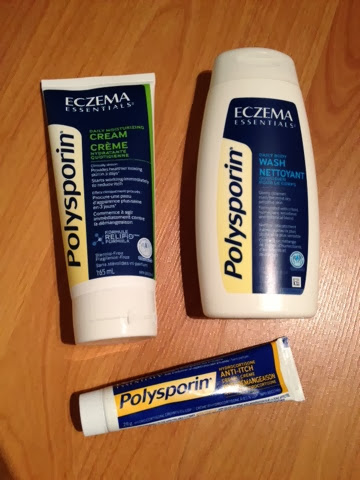The image depicts three different containers of Polysporin products designed for eczema care, all placed against a medium brown table or counter. On the left is a tube labeled "Eczema Essentials," a Polysporin product, with its logo displayed vertically in blue letters on a light yellow background. This tube is a cream, as indicated by the green text that says "cream" and "crème," with "daily moisturizing" written above it. The next item is another "Eczema Essentials" product, a daily wash bottle with similar vertical Polysporin branding on the left side. It includes the term "nettoyant" in French and some additional, albeit illegible, white text. Positioned below these two items is a smaller tube of Polysporin anti-itch cream, featuring the same color scheme of white, blue, and light yellow. Each product shares consistent branding elements, signifying different versions and uses within the Polysporin eczema care range.